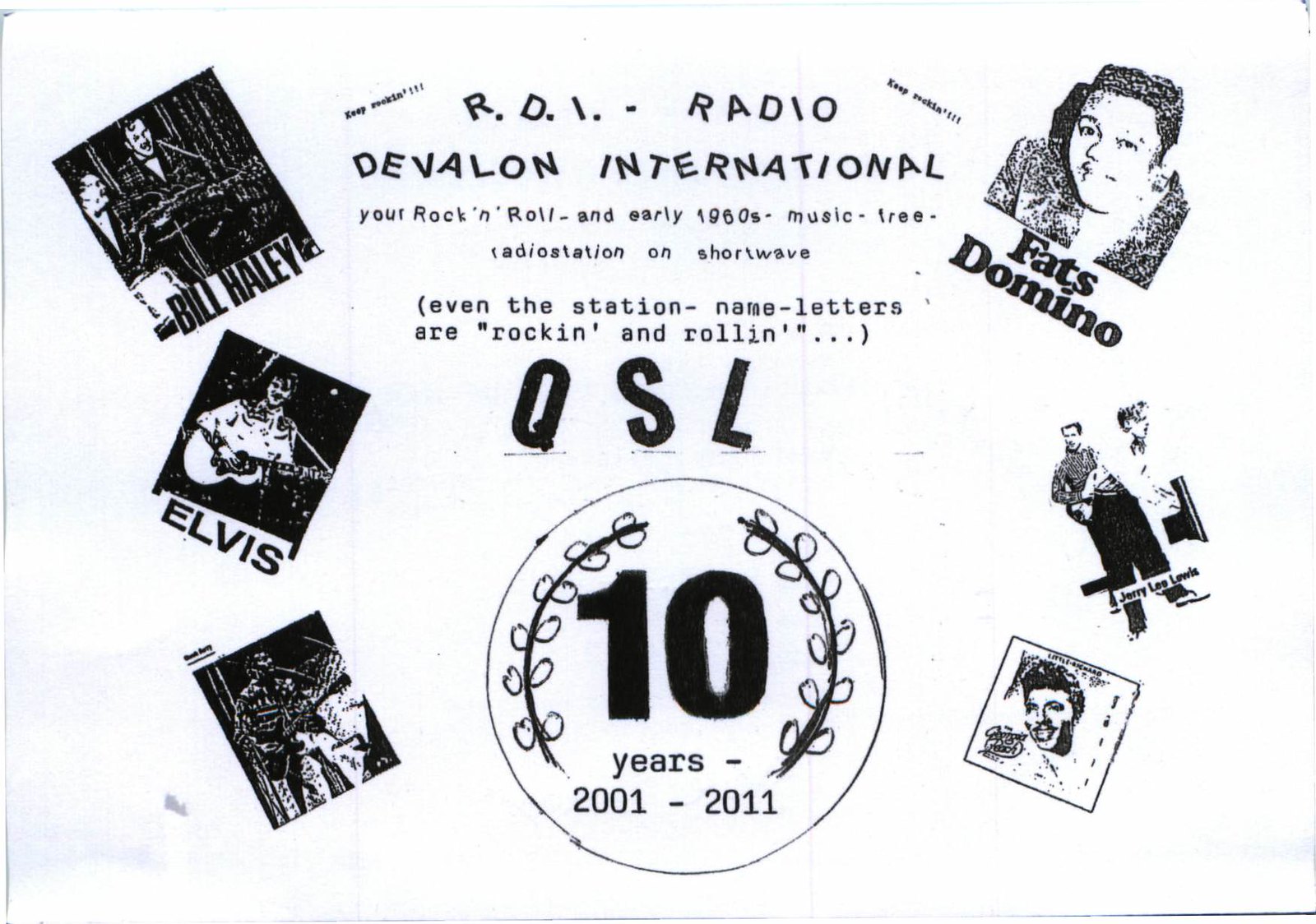This is a highly detailed poster dedicated to RDI Radio, also referred to as R.D.I. Radio Dev Vilon International, celebrating their 10 years of broadcasting from 2001 to 2011. The poster serves both as an advertisement and a commemorative graphic for this shortwave radio station known for playing rock and roll and early 1960s music. The title "R.D.I. Radio Dev Vilon International" is prominently displayed in bold characters at the top, with some letters whimsically tilted to embody the tagline: "Even the station name letters are rockin' and rollin'." 

Below the title, the term "QSL" is showcased in a large, bold font next to an image of a circular wreath pattern with a boldly inscribed '10' in the center, symbolizing the decade of their musical journey. The poster features black text on a white background and is bordered by iconic images of legendary rock and roll figures such as Bill Haley, Elvis Presley, Fats Domino, Jerry Lee Lewis, Little Richard and others. Each image is carefully placed with three musicians on the left and three on the right, although not all names are fully legible. This visually compelling montage highlights the rich heritage of rock and roll that RDI Radio has celebrated and shared with its listeners over the years.